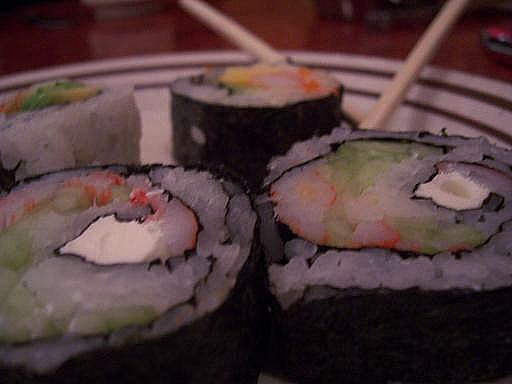This is a close-up, slightly out-of-focus image of four pieces of sushi on a white plate with two black stripes along its edge. The image captures two large sushi pieces prominently in the bottom half, featuring white rice, green cucumber, reddish-white crab or possibly shrimp, and a blob of cream cheese, all wrapped in black seaweed. The other two sushi pieces are positioned towards the back left side of the plate; one has the same seaweed wrapping while the other has rice on the outside, with yellow accents instead of white. The wooden, glossy table in the background subtly frames the white plate. Two light brown chopsticks crisscross in the background, adding to the aesthetically pleasing arrangement.